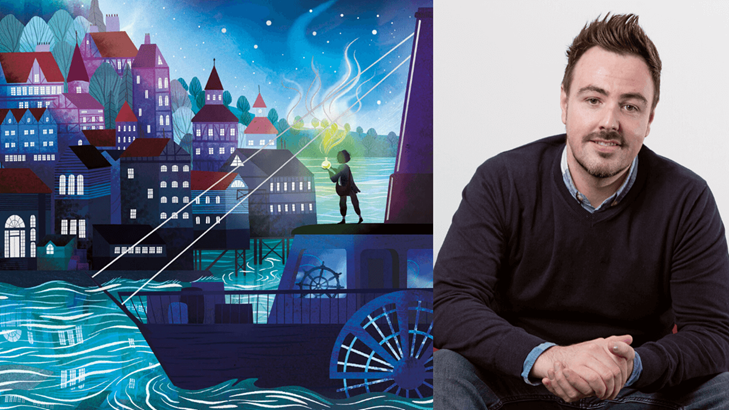A man sits on the right side of the image, appearing to be in his late 30s or early 40s. He has short brown hair styled upwards, brown eyes, and a mustache. His gentle smile and calm demeanor are accentuated by his clasped hands. Dressed in a dark shirt layered over a blue polo, he is comfortably seated and gazes directly at the camera.

To his left is a vibrant, cartoonish painting depicting a nighttime scene. The colorful artwork is rich in hues of blues, purples, and reds. The landscape features a series of houses and trees on the left, some crowned with red rooftops, overlooking a turquoise river with white reflections. This river, positioned on the right, hosts a steamboat shaded primarily in purples and blues. Atop the boat stands a child-like figure holding a yellow vial or lamp, from which yellow wisps emanate. The night sky above is dark blue, sprinkled with shimmering stars, creating a whimsical and serene atmosphere. In the background, a town with an array of multicolored buildings rises against a backdrop of green trees and distant mountains.